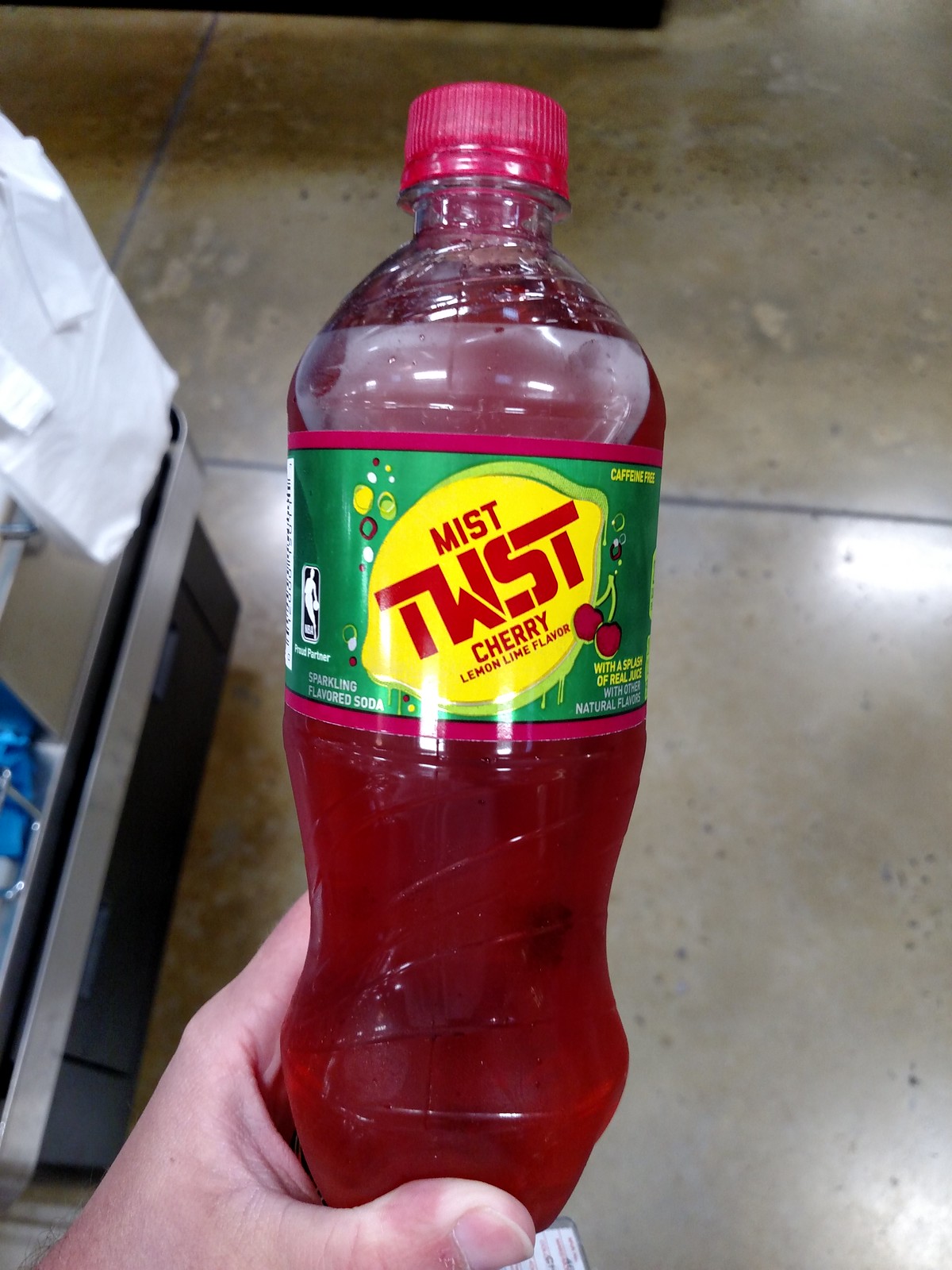In this detailed image, a person is holding up a bottle of MistTwst Cherry Lemon Lime Soda. The soda is described as caffeine-free and infused with a splash of real juice alongside other natural flavors, making it a refreshing sparkling beverage. The bottle itself is clear, revealing the vibrant red color of the drink inside. The packaging features a bright green label that prominently displays the MistTwst brand name, with "Twst" creatively spelled as "T-W-S-T" and highlighted for emphasis.

The label also showcases the flavor description in bold red lettering, nestled within an illustration of a lemon. Off to the left side of the lemon, two cherries are depicted, attached to a single stem, with one cherry partially outside the lemon graphic. This visual highlights the cherry component of the drink. Atop the bottle is a striking red cap, adding to the overall color theme of the beverage.

The background suggests the setting is a store, identifiable by the smooth laminated flooring visible in the scene.